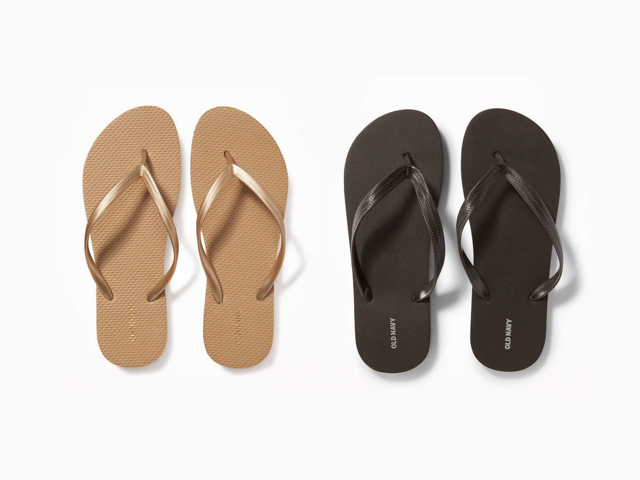The image shows two pairs of flip-flops from a top-down view on a pale background. The left pair is a taupe or tan color with shiny golden-tan straps that form a single loop attaching at the base. The right pair is black with shiny black straps of the same design. The black flip-flops have "Old Navy" written in white text near the heel, while the taupe pair also has text, but it blends with the flip-flop color making it difficult to read. Both pairs sit close together, casting slight shadows, particularly from the straps.